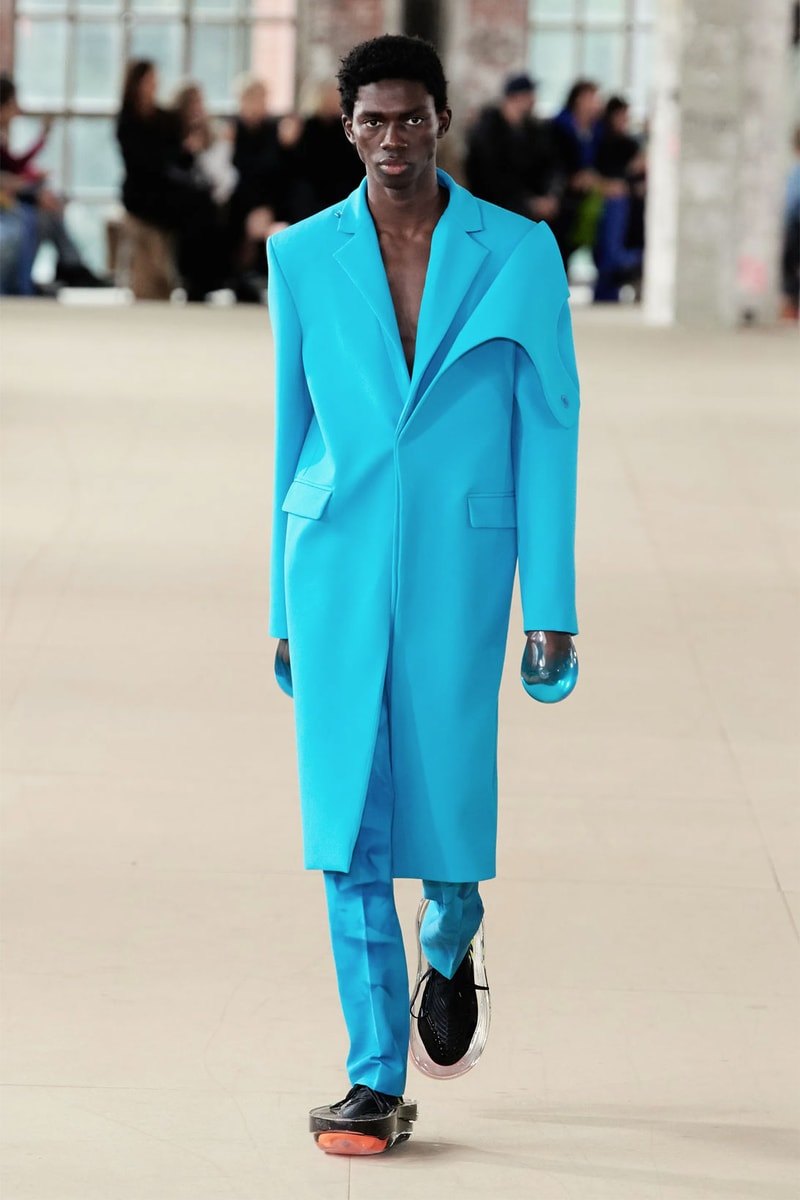This is a detailed color photograph capturing a male model in mid-step, walking confidently down the runway with a blank, serious expression on his face. The model, a dark-skinned African-American man with a short afro, exudes poise as he faces the camera directly. He is clad in a striking, turquoise blue coat that extends down to his knees, exposing his bare chest through its low-cut front. The structured style of the coat aligns perfectly with his matching narrow blue pants. Enhancing the uniqueness of his ensemble, he wears peculiar gloves adorned with clear blue, bubble-like gloves, revealing his hands inside. On his feet are distinct black shoes, each featuring an oversized, clear plastic platform. The background reveals a blurred audience, fixated on the runway, with the ground he treads being a pale tan color, complementing the cream and white hues of the backdrop.